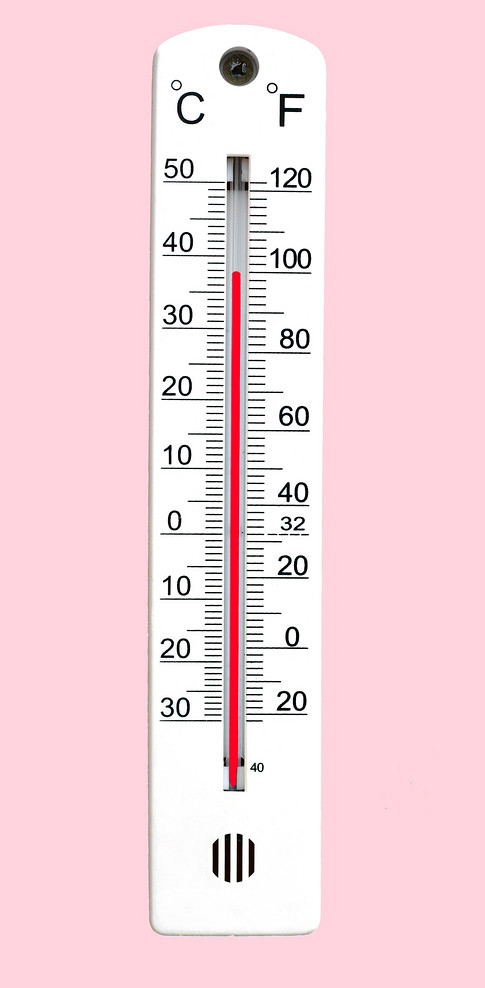This is an illustration of a thermometer set against a light pink background. The image is vertically oriented, with the thermometer prominently displayed in the center. The thermometer features dual scales for temperature measurement: Celsius on the left and Fahrenheit on the right. The Celsius scale starts at the top with 50°C and descends to -38°C. Correspondingly, the Fahrenheit scale begins at 120°F and goes down to -20°F. A thin red line runs vertically through the middle, indicating the current temperature. At the base of the thermometer, there's a circular area with white slats, resembling a speaker grille. Positioned at the top of the thermometer between the Celsius and Fahrenheit symbols is a black circle, potentially representing a screw, adding a hint of utility to the design. The entire illustration is characterized by a flat, textureless appearance with extremely even lighting, giving it a vector art aesthetic rather than the depth and texture of a photograph.